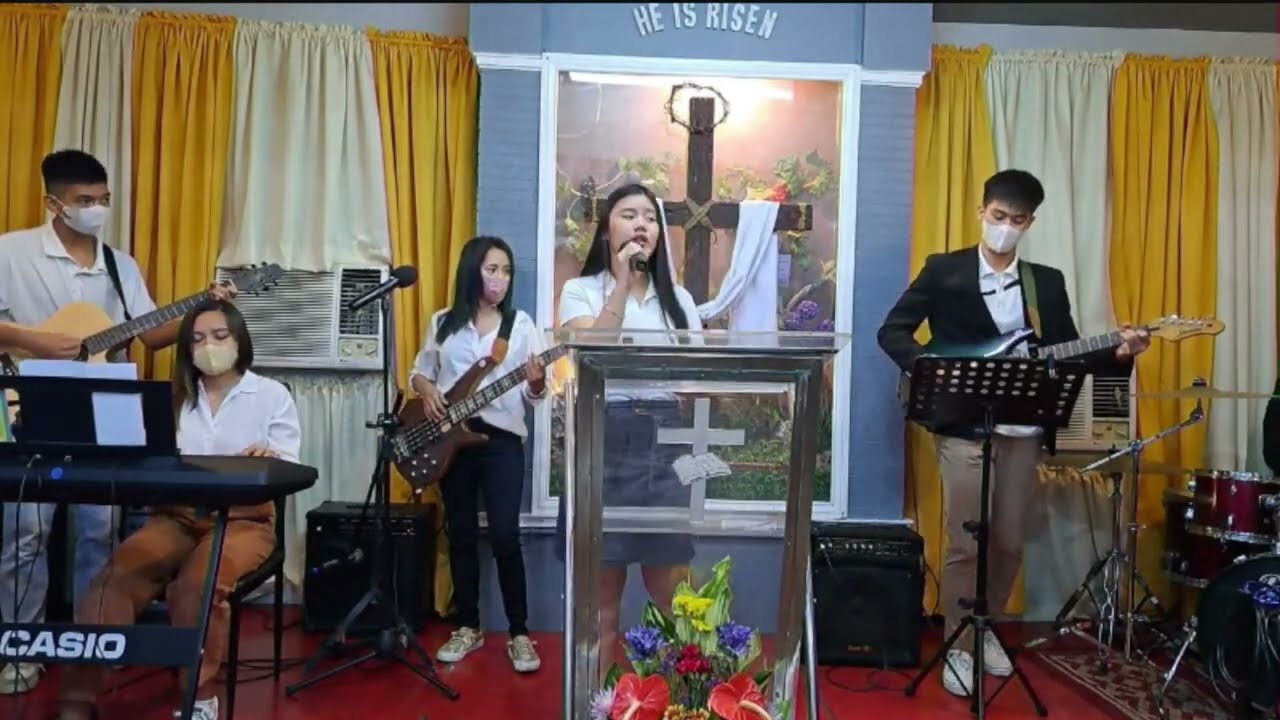The photograph captures a live religious musical performance in a quaint, small church during the COVID era, evident by the face masks worn by all performers except the singer. The church's interior is decorated with yellow and white curtains covering the windows, an air conditioner sticking out from one of them, and a distinct backdrop featuring a wooden cross adorned with a white shawl and a crown of thorns. Above the cross, set within a blue archway, are the words "He is Risen," illuminated by dramatic lighting and surrounded by flowers, with some vegetation visible behind glass. 

Center stage, a young woman with long dark hair sings into a microphone. She wears a white top and a blue skirt, standing behind a glass pulpit etched with a cross and a Bible, and adorned with colorful flowers. Flanking her are four other performers of Asian descent, all in their late teens to early twenties. To her right, a young man in a black jacket over a white button-up shirt and khaki pants plays a blue electric guitar, standing next to a set of drums. To her left, another young woman with dark pants and a white shirt plays a red electric guitar. Further left, yet another young woman, seated and dressed in a white button-down shirt and brown pants, plays a black keyboard. Completing the ensemble, a young man stands behind her, playing an acoustic guitar. The image exudes a serene yet vibrant atmosphere, embodying a moment of communal worship and musical expression.